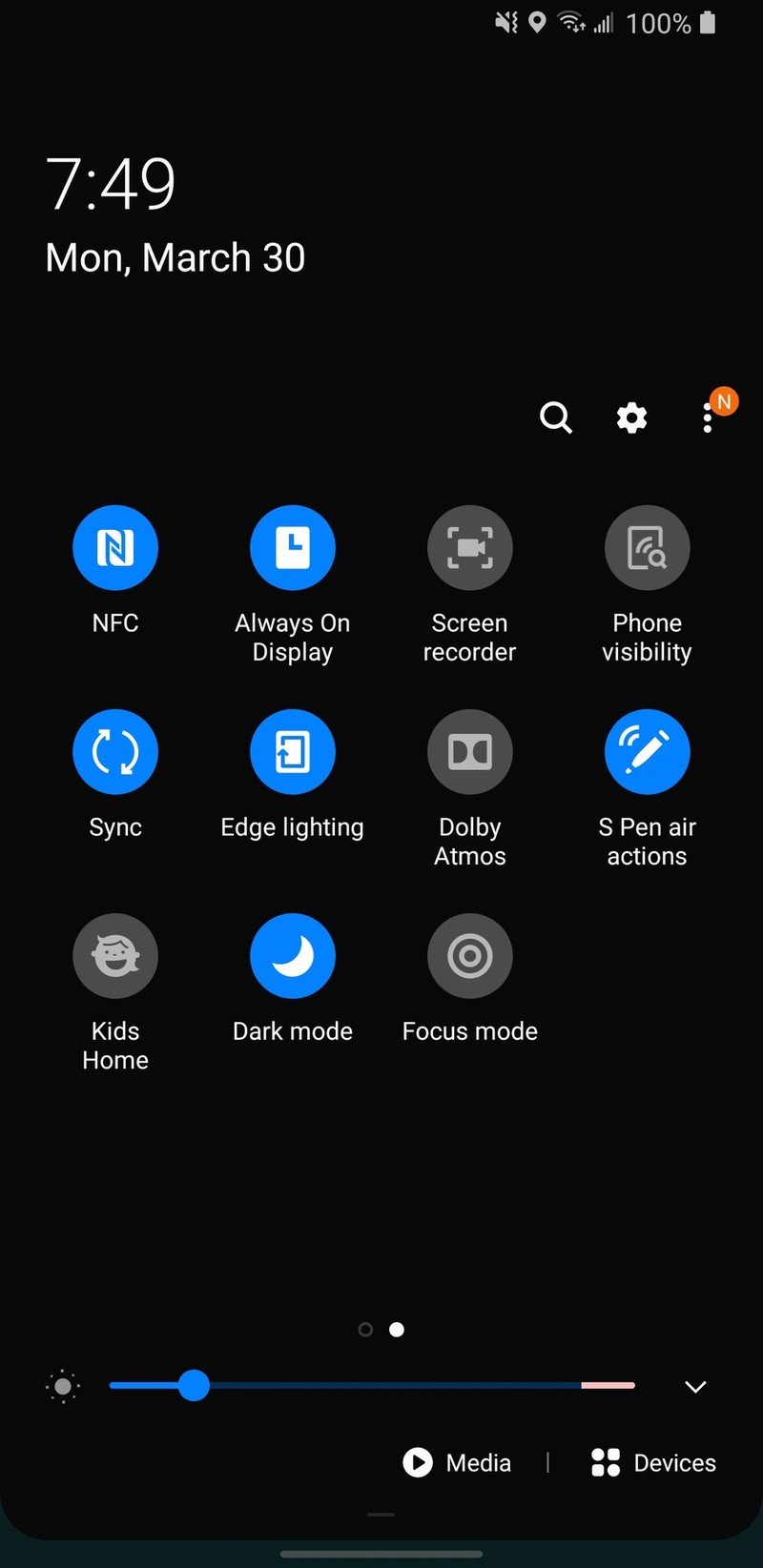Screenshot Caption: Detailed View of Phone Settings

The image showcases a screenshot of a phone's settings page, set against a deep, dark black background with white text and various icons. At the top of the screen, the phone's signal strength is displayed, showing four out of five bars. The battery is fully charged at 100%, indicating the device is at full capacity. The top left corner displays the current time, 7:49 AM, along with the date, Monday, March 30th.

The settings are organized in three rows of icons, exhibiting a mix of blue and gray circles. The first row consists of four icons from left to right: NFC (blue circle), Always On Display (blue circle), Screen Recorder (gray circle), and Phone Visibility (gray circle). The second row contains five icons: Sync (blue circle), Edge Lighting (blue circle), Dolby Atmos (gray circle), S Pen Air Actions (blue circle), and Kids Home (gray circle). The third row includes Dark Mode (blue circle) and Focus Mode (gray circle).

At the bottom of the settings page, there are two additional options labeled "Media" and "Devices." A prominent blue slider runs from left to right at the very bottom, adding to the overall navigational aids presented on the screen. The combination of blue and gray icons provides a clear visual distinction between different settings, enhancing the user experience.